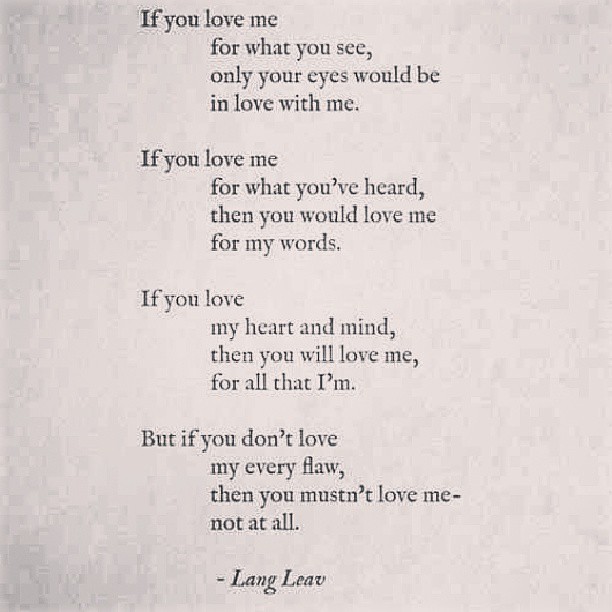The image showcases a poem on a light purple or off-white background, featuring black text elegantly laid out in four small, centered paragraphs. The poem reads: “If you love me for what you see, only your eyes would be in love with me. If you love me for what you've heard, then you would love me for my words. If you love my heart and mind, then you will love me for all that I am. But if you don't love me, my every flaw, then you mustn't love me, not at all.” The repeated phrase, "If you love me," is offset slightly to the left in each stanza, creating a visually appealing flow. At the bottom, the author’s name, Lang Leav, is clearly displayed, attributing this thoughtful and poignant piece to the well-known poet.